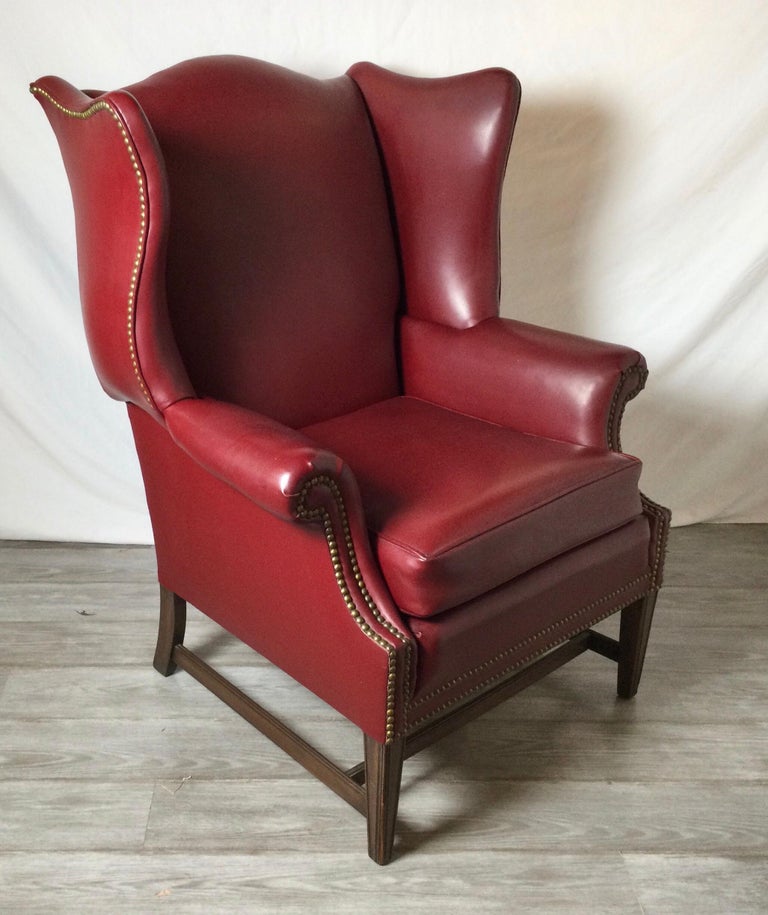The image showcases a close-up of a luxurious armchair bathed in vibrant maroon-red hues, resembling either leather or high-quality pleather with a glossy finish that gleams under the light. The chair's standout design features include rolled arms and winged side panels extending upwards from the headrest, all meticulously adorned with brass or gold-colored tacks forming a dotted trim along the armrests, side panels, and chair base. The armchair's sturdy legs and undercarriage are crafted from rich, dark wood, and are interconnected by horizontal support bars, ensuring stability. This elegant piece rests on a light grayish, wood-patterned floor, set against a backdrop of beige or white fabric, creating a minimalist yet sophisticated scene. The harmonious blend of textures and colors, from the maroon leather to golden accents and wooden elements, culminates in a refined and striking visual composition.